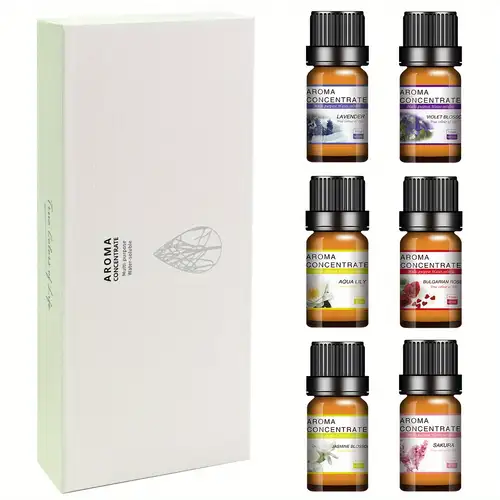This image showcases a set of six aroma concentrate bottles positioned on the right-hand side. The bottles are arranged in three rows with two bottles in each row, next to a white rectangular box labeled "Aroma" with a gray leaf design. Each of the six round amber bottles with black lids bears the "Aroma Concentrate" label and feature different colored labels: the top row consists of blue and purple bottles, the middle row includes yellow and red bottles, while the bottom row displays yellow and pink bottles. The scents appear to be lavender, violet blossom, aqualette, lemon, raspberry, and a green flowery substance, though some labels are not entirely visible. The box likely contains the bottles and serves as the product packaging.